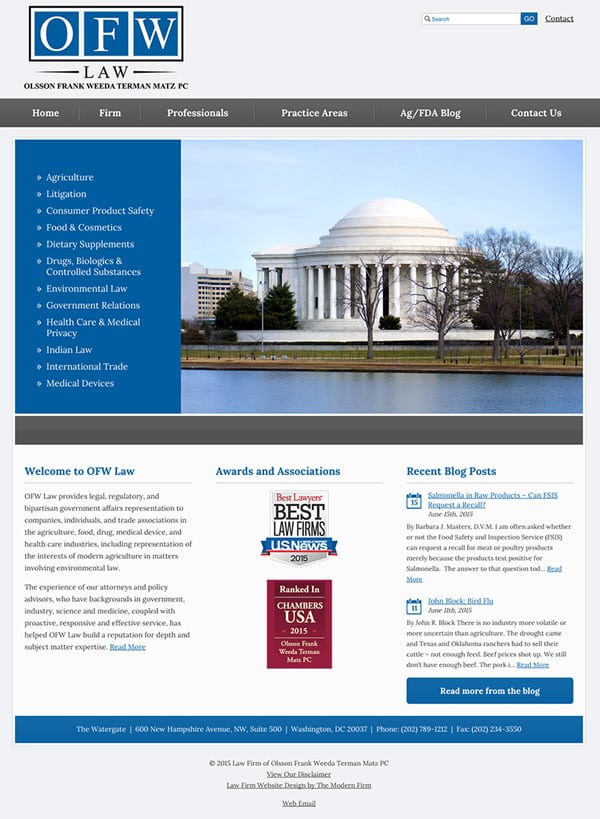Screenshot of a Law Firm Website:
 
In the upper left-hand corner, the logo of OFW Law is prominently displayed with three blue boxes containing white text that says "OFW". Below this, in black text, it reads "Law," and further down in smaller black text, it states "Olson, Frank, Weta, Thurman, Max, PC." Adjacent to this logo setup, in the upper right-hand corner, a search bar is positioned, followed by a blue button with white text, and to the right is the word "Contact."

Beneath the header section, there’s a gray navigation bar with white text offering different headers: "Home," "Firm," "Professionals," "Practice Areas," "AG," "FDA," "Blog," and "Contact Us." Directly below this navigation menu, on the left side, appears a blue box featuring several bullet points labeled comprehensively, including "Agriculture," "Legislation," "Consumer Product Safety," "Food and Chemicals," "Dietary Supplements," "Drugs," "Biologicals," "Controlled Substance," "Environmental Law," "Government Relations," "Healthcare," "Medical Practice," "Indian Law," "International Trade," and "Medical Devices," all in white text.

To the right of this blue box is a striking image of a white domed building adorned with numerous columns encircling its structure. In the foreground, a serene blue river snakes along, bordered by several trees devoid of leaves. The background of the picture showcases a clear blue sky.

Below this image, there's an empty gray bar, followed by three distinct columns beneath it. The first column, titled "Welcome to OFW Law," presents an introduction to the law firm. The middle column, labelled "Awards and Association," displays two plaques, indicating recognitions such as "Best Law Firm,” US News, and “Ranked in Chambers USA 2015.” The third column, "Recent Blog Posts," features entries of two recent blog posts from the firm.

This detailed layout provides a comprehensive insight into the content and visual elements present on the captured screenshot of the law firm’s website.